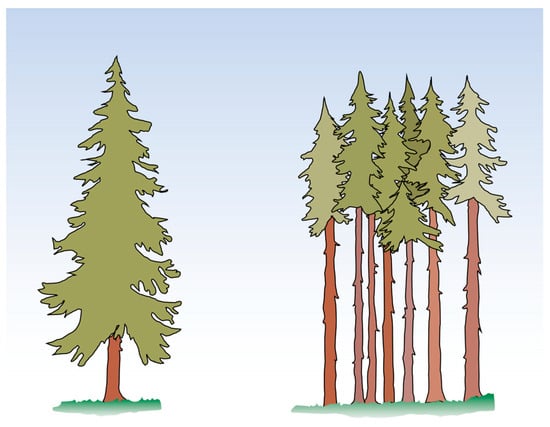This is a simple, two-dimensional rectangular image, slightly wider than it is tall, resembling clipart or a basic computer drawing. The background features a linear gradient, starting with a light sky blue at the top and fading seamlessly into white at the bottom. The bottom left of the image holds a small patch of green grass with a single, tall evergreen tree with a prominent brown trunk and green foliage at the top. On the bottom right, there's a larger patch of grass supporting seven thinner evergreen trees, each with disproportionately tall brown trunks and green foliage condensed at the very top. The foliage for these trees starts much higher up, giving the impression of missing middle sections. The image's overall aesthetic is flat and straightforward, with clear outlines and no additional shading beyond the background gradient.